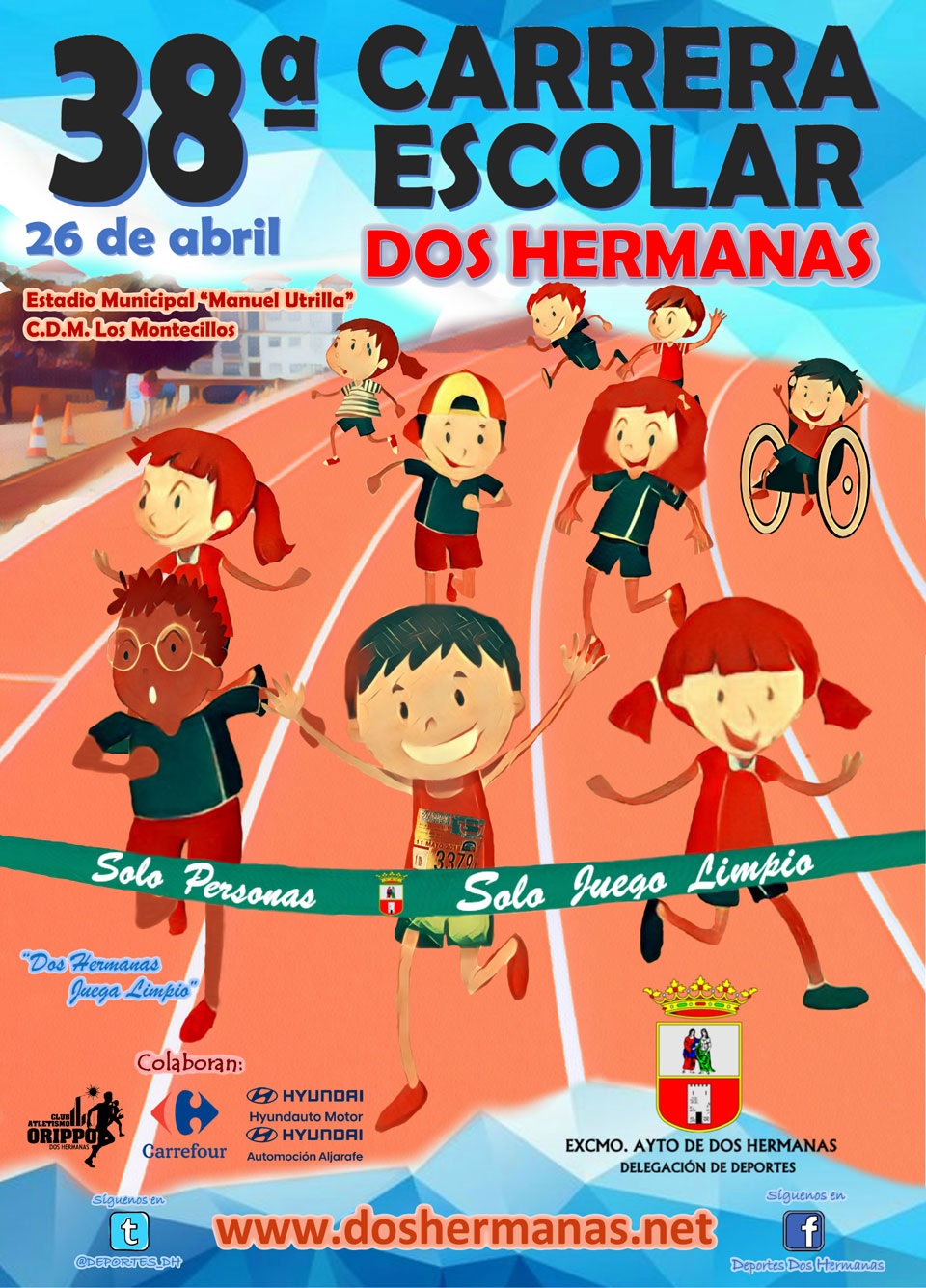The image showcases a colorful poster for the "38A Carrera Escolar Dos Hermanos," a school race event. Set against a blue sky background, the poster features vibrant, computer-illustrated children, including boys, girls, and one boy in a wheelchair, energetically running on an orange racetrack marked with white lane lines. The group of nine children is organized in rows of three, all smiling and participating in the race. A green banner with the phrases "solo personas, solo juega, limpio. Solo juega, limpio" in white text stretches across the front of the runners. The upper left-hand corner bears the black number "38" alongside an underlined letter "A", indicating the event's edition. The name "Carrera Escolar Dos Hermanos" is prominently displayed in red letters next to it. Below the track, a blue geometric area frames various advertisements, including brands like Hyundai and Facebook. At the very bottom of the poster, the event's website, "www.doshermanos.net," is written in orange letters.